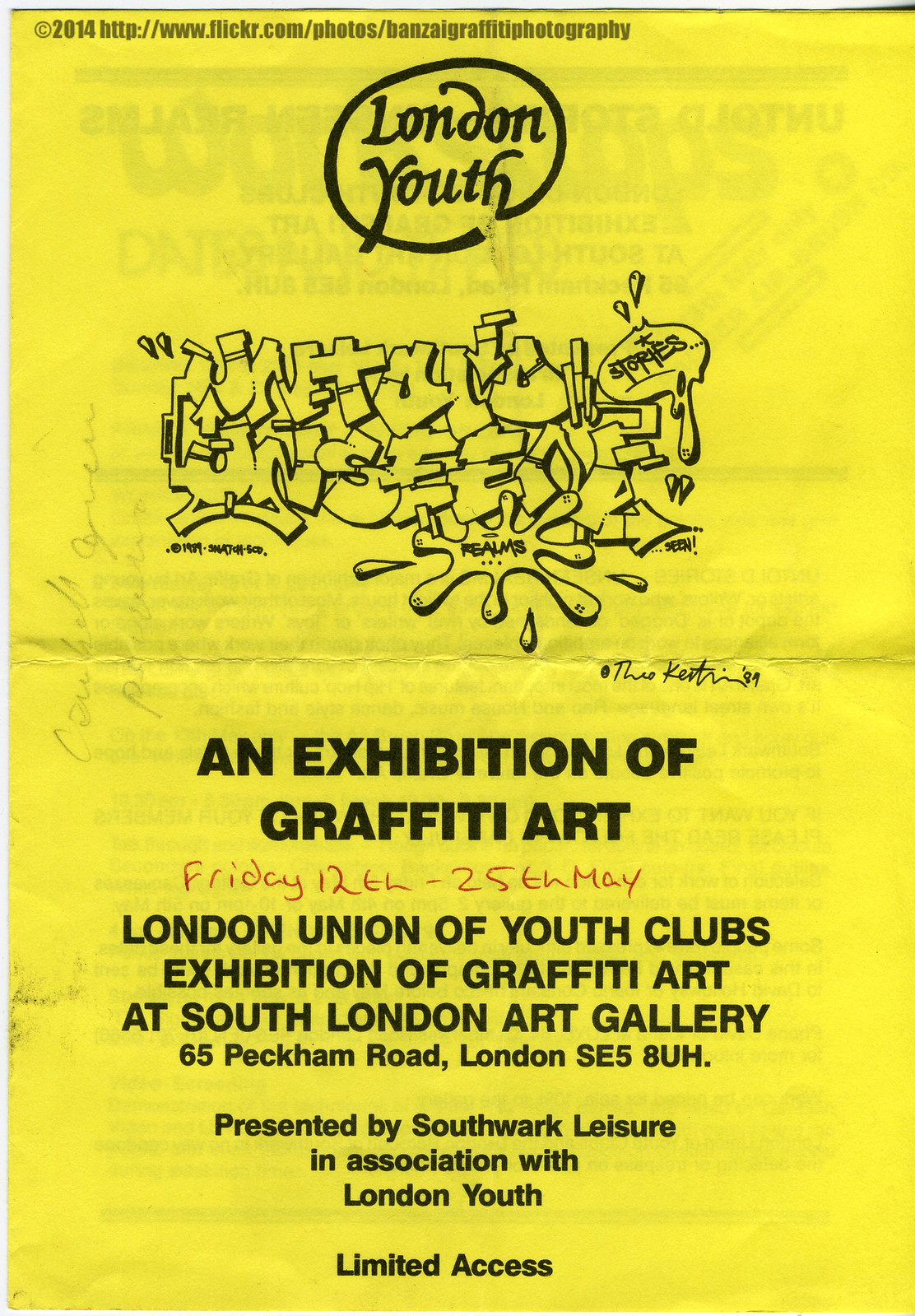The image displays a yellow flyer, reminiscent of a magazine page in dimension, featuring rich visual and textual details in black, white, and red. Centered prominently at the top, the headline reads "London Youth," encircled in black. Above it, on the upper left corner, "2014" and a URL, "http://www.flickr.com/photos/BanzaiGraffitiPhotography," indicate the source. Dominating the midsection, an outlined illustration of graffiti art separates the headline from the event details. Below the graffiti, bold text announces "An Exhibition of Graffiti Art," followed by red handwritten dates, "Friday 12th to 25th May." The flyer further details the event hosted by the London Union of Youth Clubs at South London Art Gallery, located at 65 Peckham Road, London SE5 8UH. The flyer concludes with "Presented by Southwark Leisure in association with London Youth Limited Access," emphasizing the collaborative and restricted nature of the event. The flyer, noticeably creased from a past fold across its center, captures attention with its striking use of color and urban artistic theme.